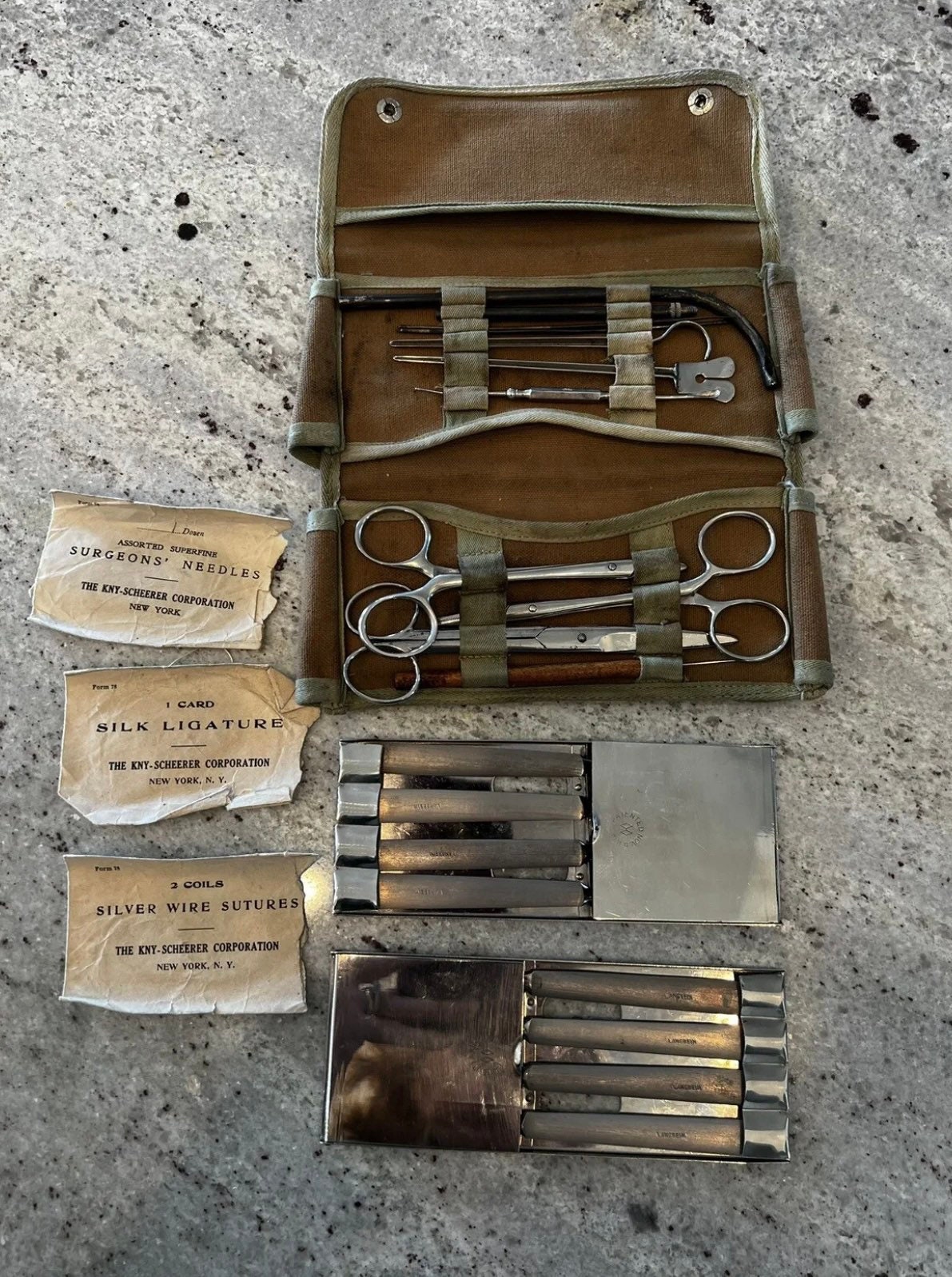The image depicts a close-up of an old surgical toolkit, likely used by a doctor for house calls. The tools are meticulously arranged within a worn, leather-bound duffel bag. Notably, there are silver surgical instruments including two pairs of scissors, tweezers, syringes, and various other implements such as hooks and scraping tools, potentially for dental or surgical procedures. Among the items are multiple silver trays containing rectangular objects. Scattered papers label these implements, detailing their uses: one card labeled "Assorted Superfine Surgeon's Needles" from the KNY, Schroeder Corporation, New York, a second card reading "Silk Ligature," and a third for "Silver Wire Sutures." The labels and tools rest on what appears to be a gray, marble countertop.